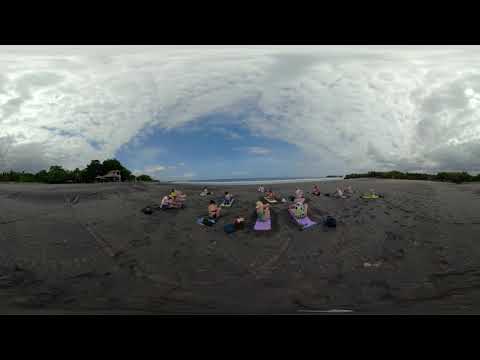In this outdoor daytime photograph, there is a group of around 12 to 13 people sitting on beach blankets in a semicircle on what appears to be dark gray sand or dirt. The image is somewhat blurry, making it difficult to distinguish precise details, yet the sand seems to be marked with ruts and footprints. The scene is framed by black rectangles at the top and bottom. The background features rows of trees on either side, with an opening that suggests a lake or sea outlet further off. There is a house visible on one side, surrounded by numerous trees, while the rest of the scenery is dominated by more trees and possibly mountains in the distance. The sky is mostly cloudy, covering about 80% of it, but a half circle of blue sky opens up right above where the people are sitting. This makes for a scenic backdrop amidst the natural surroundings.